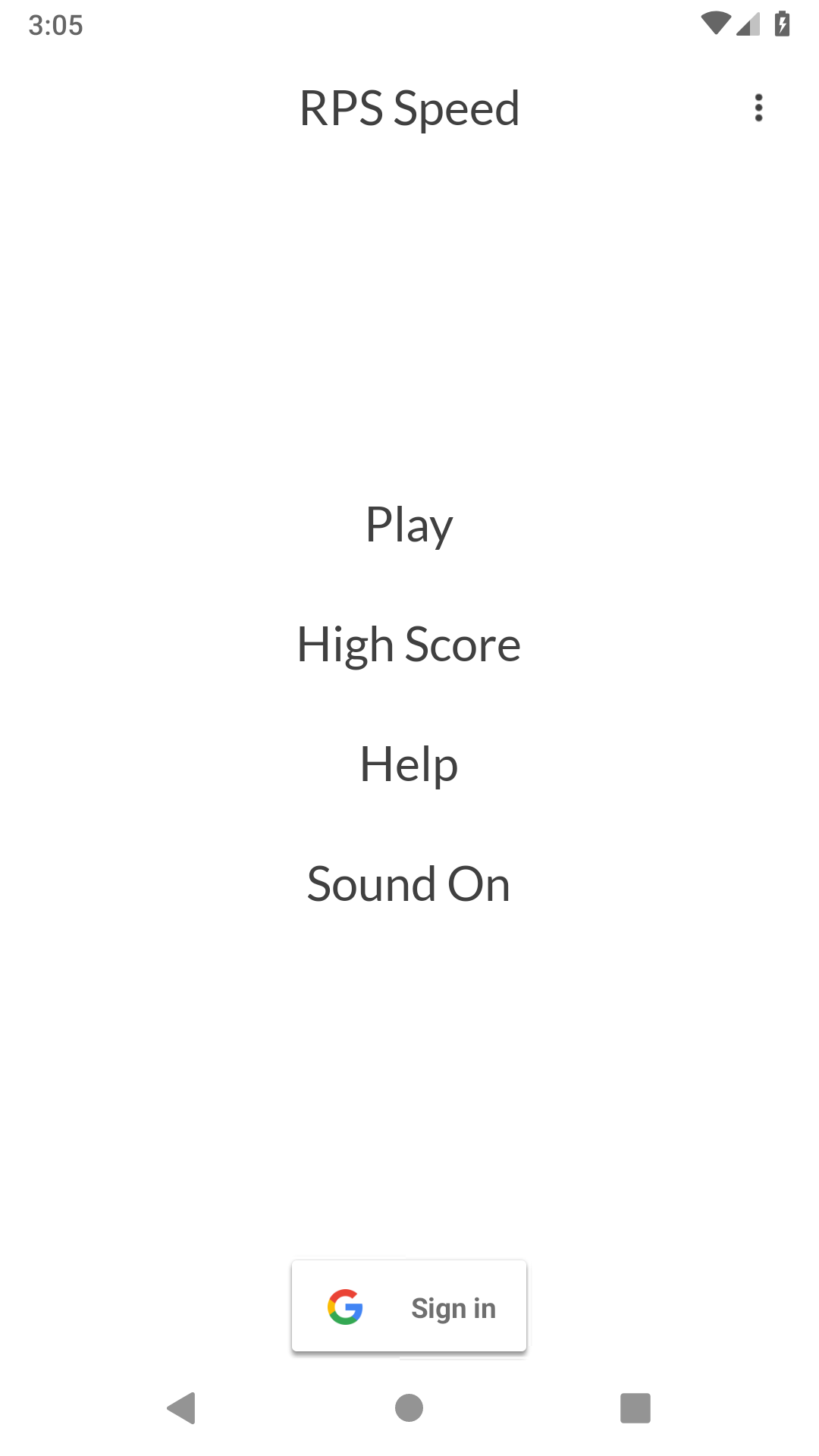The image is a screenshot taken from a phone. In the top left corner, the time is displayed as 3:05. Moving to the top right corner, the phone shows a full Wi-Fi signal icon, a signal strength indicator with 2 out of 4 bars, and a battery icon. Centrally positioned below this, in capital black letters, are the words "RPS" followed by "Speed" with a capital "S" and lowercase "peed" below it. 

After skipping several lines, four centered options are listed, each starting with a capital letter: "Play," "High Score," "Help," and "Sound On." Below these options, there is a white rectangle with a dark grey border that features the Google "G" logo on the left side and the words "Sign in" on the right. Positioned beneath this rectangle are three dark grey symbols: a left-pointing arrow, a circle, and a square.